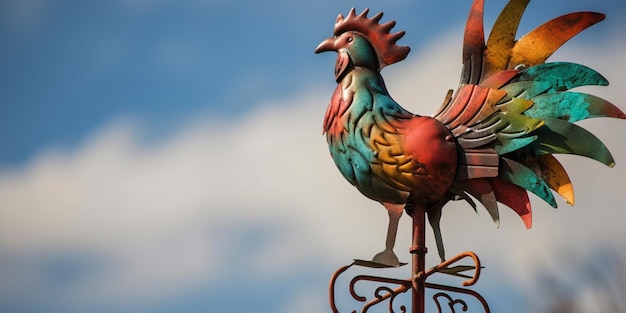The image is a highly detailed and realistic photograph of a vibrant metal rooster weather vane set against a daytime sky marked by light blue hues and scattered white clouds, dominated by one large, fluffy white cloud. The weather vane, prominently featured in the center of the image, stands atop a light brown pole adorned with four small hooks. The rooster itself is a kaleidoscope of colors: burnt red-orange, teal blue, green, and bright yellow. It has a striking red comb atop its head and a richly adorned chest in reds, blues, and yellows. Its tail feathers, resembling those of a peacock, are a mix of reds, blues, greens, and yellows, giving it a vibrant and dynamic appearance. The intricate metal layers and decorative swirls at the base of the vane add to the artistic aesthetic, making the rooster a focal point of both visual interest and function, guiding directional winds.